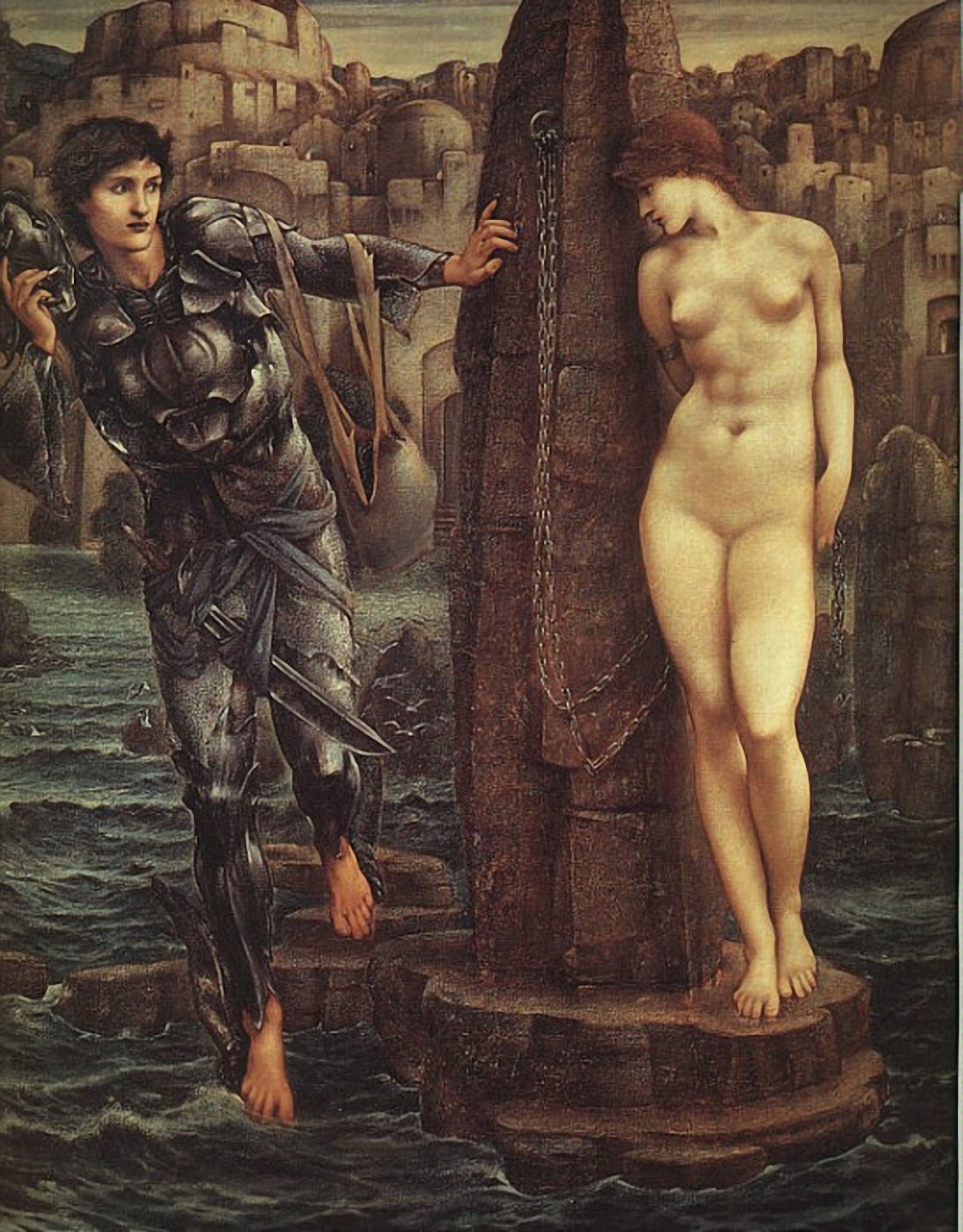The image showcases a painting depicting a mythological scene set amidst a turbulent waterway. The foreground features two prominent figures: a barefoot woman and a knight-like man. The woman, positioned on the right, stands naked with her left arm adorned with a chain connected to a stone pillar. She has long, reddish-braided hair and gazes toward the left. The stone pillar she leans against is part of a rocky islet surrounded by choppy waters. The man on the left, with dark hair, wears a grey, armor-like garment that appears softer than typical armor. He holds a helmet in his right hand and has a mask in his other hand, with a rope draped over his arm. He peeks around the pillar, casting his gaze toward the woman. The background reveals a mass of grand, domed buildings, suggesting an ancient or mythological setting.